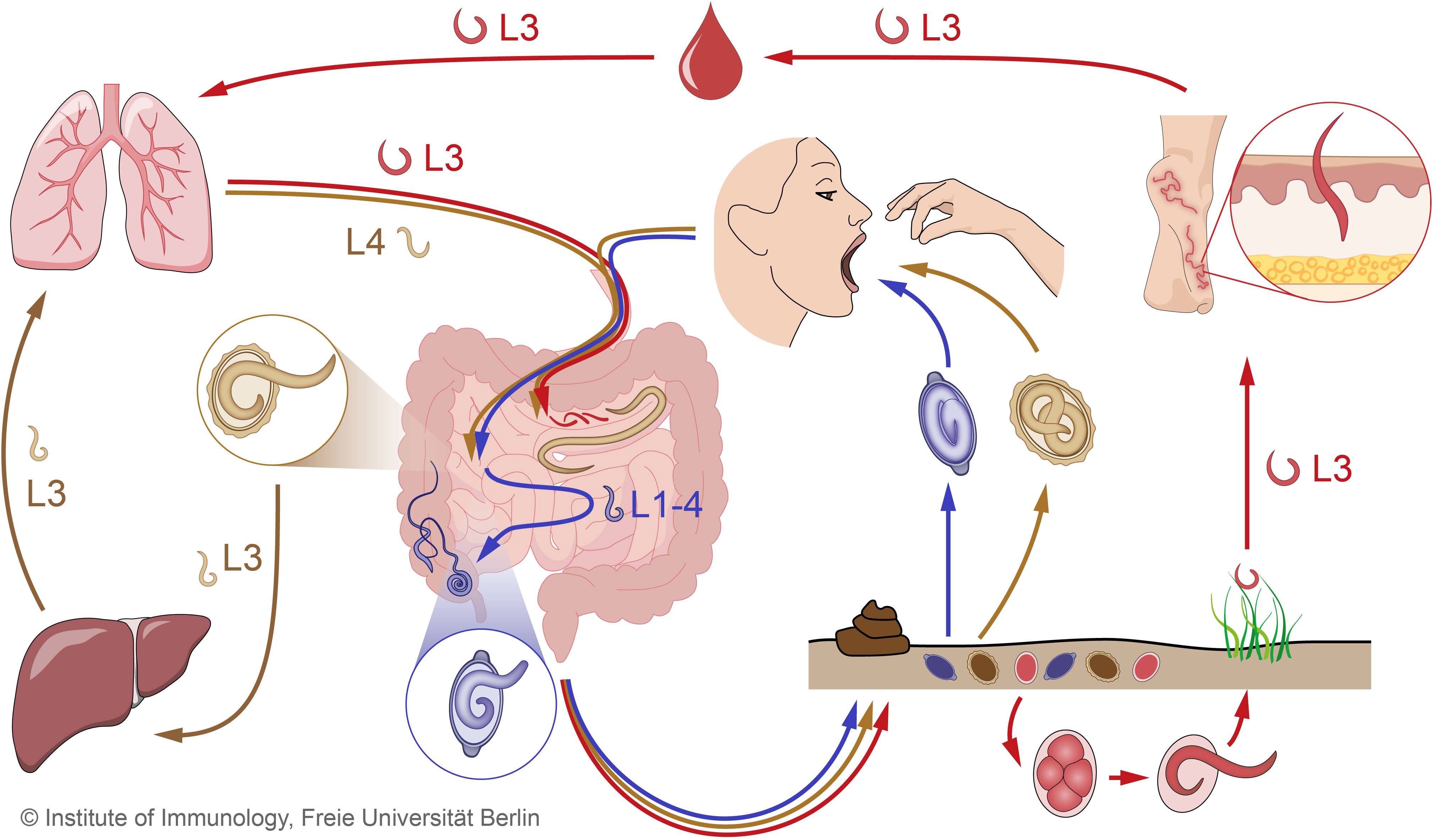This detailed diagram serves as an intricate flow chart elucidating the life cycle and bodily circulation of parasitic infestations. Central to the image is an illustration of a woman’s profile with her mouth wide open and a hand poised to place something into it. Arrows, depicted in blue and gold, trace the pathways these parasites take once introduced into the body.

Beginning in the bottom right corner, the diagram features a light brown line symbolizing soil, adorned with green grass leaves and fecal matter, highlighting the environmental origin of the parasites. The parasites themselves are depicted as a blue worm within an oval and a yellow worm within a spiky circle. These elements underscore the parasites' journey from contaminated soil into the body.

From the soil, an arrow directs attention to the woman's open mouth, symbolizing ingestion. Adjacent to her head, colored peach, further arrows denote the passage of the parasites down into the intestines. The intestines are detailed with specific lines mapping the parasites' journey, including paths towards the liver and lungs, illustrating the various organs affected by the infestation.

Additional diagrams include a detailed view of the bottom of a foot, showing a parasitic entry point at the skin layer, and subsequent arrows indicating systemic travel through the bloodstream to the lungs. The diagram also features tear-shaped and cone-shaped symbols representing different stages and forms of the parasites, with labeled lines, such as “L3,” marking critical stages of their lifecycle and highlighted points of infection.

In the top right corner, a conspicuous red circle with cream-colored skin and a red slice emphasizes another aspect of the parasite's destructive path. Meanwhile, the continuous line of the life cycle concludes with arrows returning to the soil, thus showcasing the reproduction and recontamination cycle of parasites. This comprehensive flow chart is attributed to the Institute of Immunology at the Freie University of Berlin, as noted by the text within the diagram.